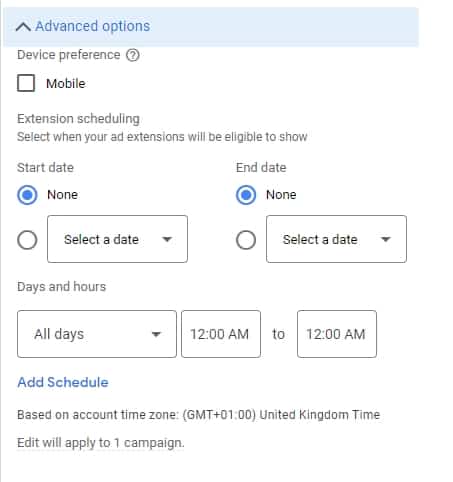Screenshot of the "Advanced Options" Section in a Website Form

The displayed screenshot is from a website form showcasing the expanded "Advanced Options" view. This section allows users to customize device preferences and scheduling settings. Key elements include:

1. **Device Preferences:**
   - A checkbox labeled "Mobile" is visible, allowing users to select if their preference pertains to mobile devices.

2. **Extension Scheduling:**
   - A text prompt instructs users to select when their extensions will be eligible to show.
   - **Start Date Options:**
     - "None" is the default selection with an accompanying radio button.
     - Another radio button is available for a "Selected Date," which is not chosen.
   - **End Date Options:**
     - Similarly, "None" is the default selection with its radio button selected.
     - Another radio button for a "Selected Date" is available but not selected, showcasing a drop-down menu option.
   
3. **Days and Hours:**
   - A drop-down menu labeled "All Days" is present allowing users to choose specific days.
   - Two adjacent fields are available for users to input specific times of day, currently set from "12:00 AM" to "12:00 AM."
   
4. **Additional Features:**
   - A link labeled "Add Schedule" is visible, enabling users to add more custom scheduling options.
   - Informational text at the bottom indicates that scheduling is based on the account time zone (GMT+0100, United Kingdom time) and will apply to one campaign.

The webpage features a clean design with black text complemented by blue highlights. A prominent blue band spans across the top, set against a white background, enhancing readability and visual clarity.